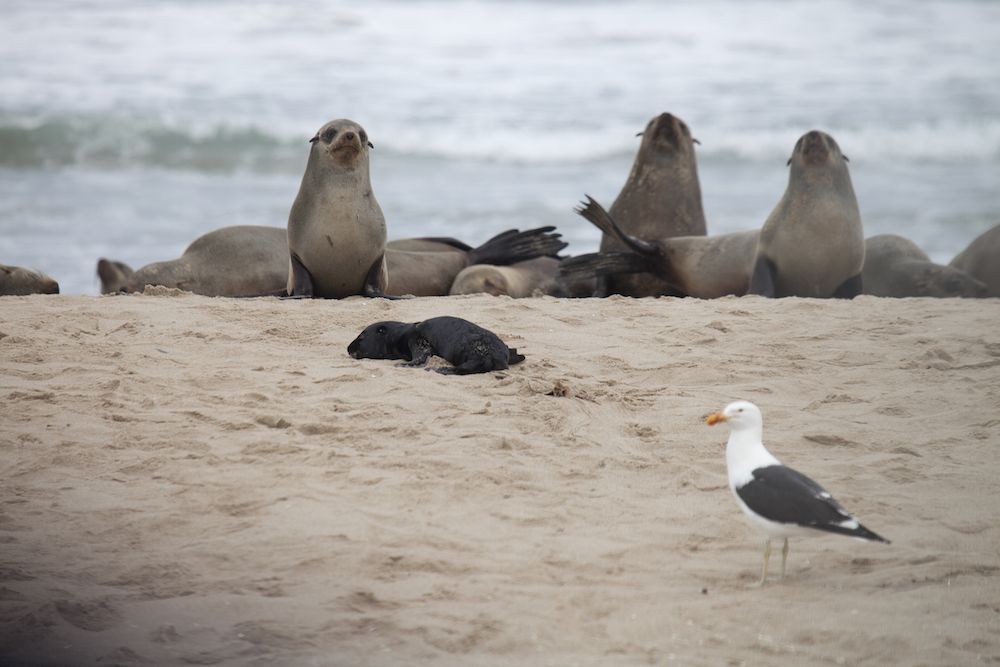This is a color photograph capturing a serene beach scene occupied by wildlife. In the foreground, a white seagull with black wings and an orange-yellow beak stands on the sandy shore, looking left. Nearby, there appears to be a dead seal pup, small and black, partially buried in the sand. In the middle distance, a group of light brown seals sprawls across the beach, with three of them alert with heads up, seemingly gazing towards the camera, while others rest peacefully. The seals exhibit darker brown flippers and tails. The background showcases the ocean, its blue waters speckled with white-topped waves, suggesting a lively surf. The colors in the image range from sandy beige, ocean blue, and varying shades of gray and brown, framed under a sunny sky.